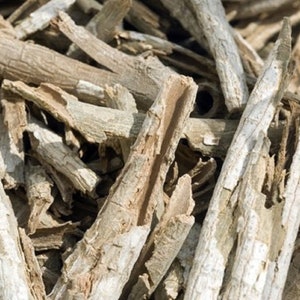The photograph is a small square image showcasing a pile of broken wood pieces, likely driftwood or remnants from fallen trees, filling the entire frame. The wood appears to be a light gray, with the peeling bark suggesting it might be from birch trees. Two large pieces dominate the foreground, extending from the bottom towards the upper right corner, revealing a dark tan interior. Surrounding these main pieces, numerous smaller branches and wood fragments point in various directions, with some angled towards the left. The bright sunlight casts shadows that obscure some parts of the wood, adding depth and highlighting the texture. The scene is suggestive of natural damage rather than mechanical cutting, giving the impression of a chaotic yet naturally beautiful arrangement.